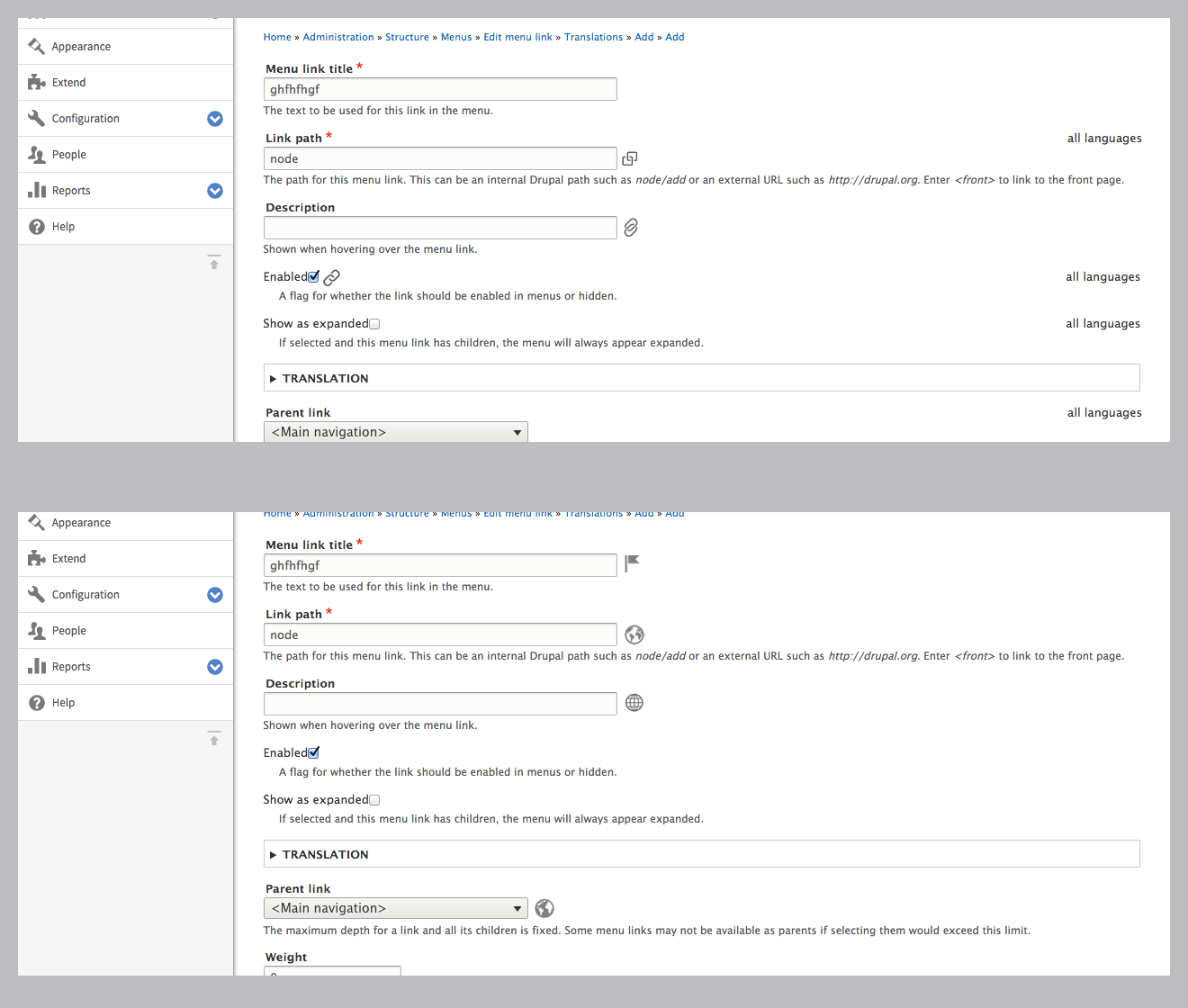The image showcases a user interface with a gray background divided into two main sections, each occupying roughly half of the vertical space. Both sections are bordered in white. 

In the top section, there is a left-hand sidebar featuring a vertical list with the following categories: "Appearance," "Configuration," "People," "Reports," and "Help," each accompanied by a corresponding icon. Notably, there are small drop-down arrows next to "Configuration" and "Reports," suggesting additional options underneath these categories. To the right of this sidebar is a form area where users can input details. The fields available for input include "Menu Link Title," "Link Path," "Description," "Enabled," "Show as Expanded," and "Parent Link." An additional label, "All languages," appears in the upper-right corner of this section, perhaps indicating language settings. 

The lower section mirrors the top section almost identically, containing the same sidebar categories, icons, drop-down arrows, and input fields for "Menu Link Title," "Link Path," "Description," "Enabled," "Show as Expanded," and "Parent Link." One distinction, however, is the absence of the "All languages" label in the lower section.

Overall, the image depicts a clear, structured layout likely meant to facilitate user interactions through a consistent, duplicated interface.